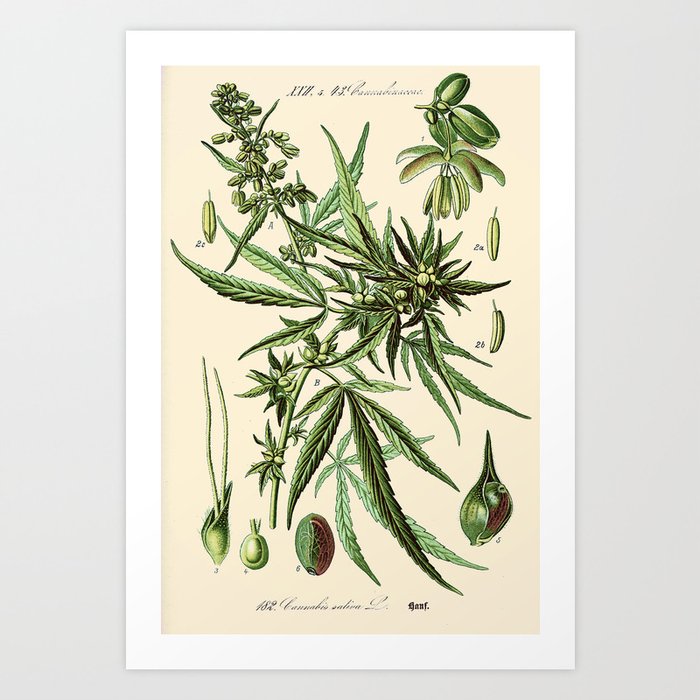This detailed botanical illustration features the cannabis sativa plant, presenting various stages and parts of its development. The image is framed with a white border and set against a tan or cream background. Notable features include thin, green, serrated leaves, which are striated and often appear in groups of five, conveying their spiky and elongated nature. Scattered around the image are detailed depictions of the plant's seeds, pistils, and male parts. Each part is carefully labeled with numbers corresponding to the botanical elements depicted, such as the small, round pods and green droplet-like structures in the bottom corners. Elegant cursive text at the top and bottom of the image provides additional botanical information, enhancing its scientific presentation. This meticulous arrangement paints a comprehensive picture of the cannabis sativa plant, encapsulating its botanical intricacies in a visually engaging manner.